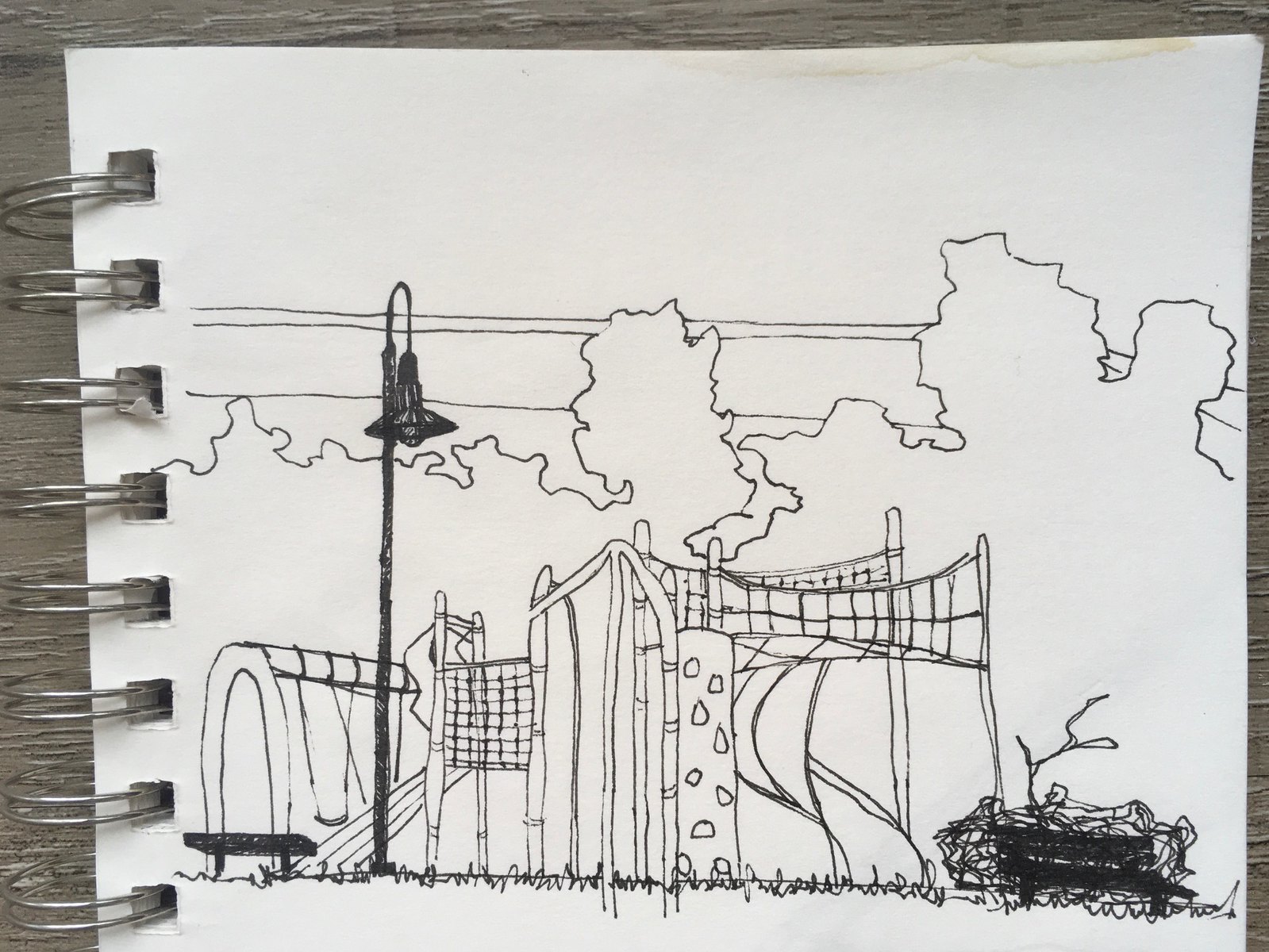This detailed black and white sketch, rendered in pen on a three-ring spine sketch pad, captures a bustling playground teeming with various play structures. The intricate drawing features a swing section prominently displayed next to a linear slide. Adjacent to the slide, a walkway enclosed by net panels adds to the playground's complex design. A cylindrical rock-climbing section seamlessly integrates with a set of monkey bars, all contributing to an obstacle course-like atmosphere. Adding to the playground's allure is a curving slide that coils within the play area, blending with nets and climbing features around it.

In addition to the playground equipment, the sketch artist also included a lamppost that subtly illuminates the scene. Overhead, clouds drift lazily across the sky, adding depth and a touch of whimsy. On the bottom right corner, a bird's nest lies on the ground, introducing a charming and unexpected element to this intricate and lively playground illustration.